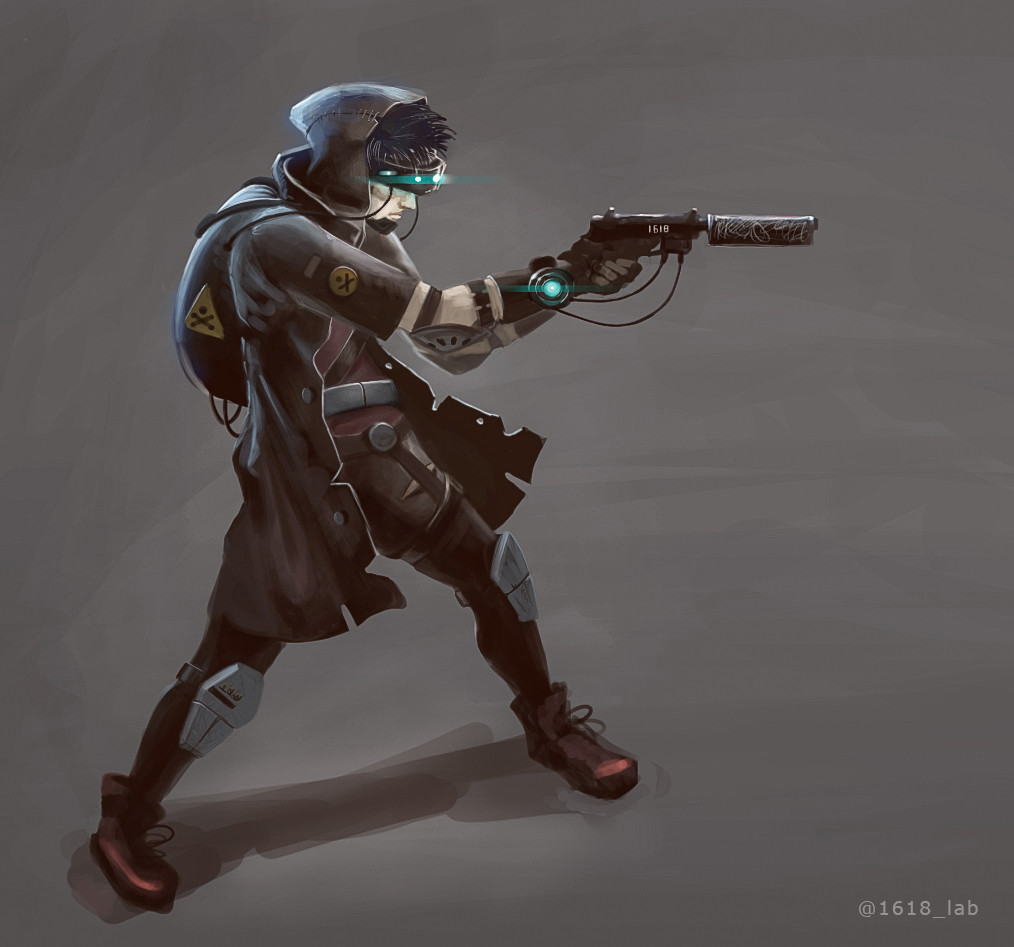The image is a highly detailed, computer-generated depiction of a video game character. The character stands against a gray, gradient background with no discernible pattern. In the bottom right-hand corner of the image, there is the text "@1618_LAB."

The character is male, with white skin and black hair, exuding a serious demeanor. He is dressed in a predominantly brown, steampunk-style outfit that includes an overcoat with a hood, which is pulled over his head, partially concealing him. His garments also include laser glasses that wrap around his head and a futuristic bracelet emitting a green light, matching the green light on his headband.

He is equipped with knee pads, elbow pads, and red laced boots, and he sports leather fingerless gloves. A drawstring backpack with a triangular hazardous materials patch is slung over his shoulder, and a similar circular patch is visible on his sleeve. His wristwatch appears more like a high-tech gadget.

The character is armed, holding a gun inscribed with "1618" and aiming it to the right-hand side of the image. He appears to be looking through the gun's scope, reinforcing his focused and serious expression.